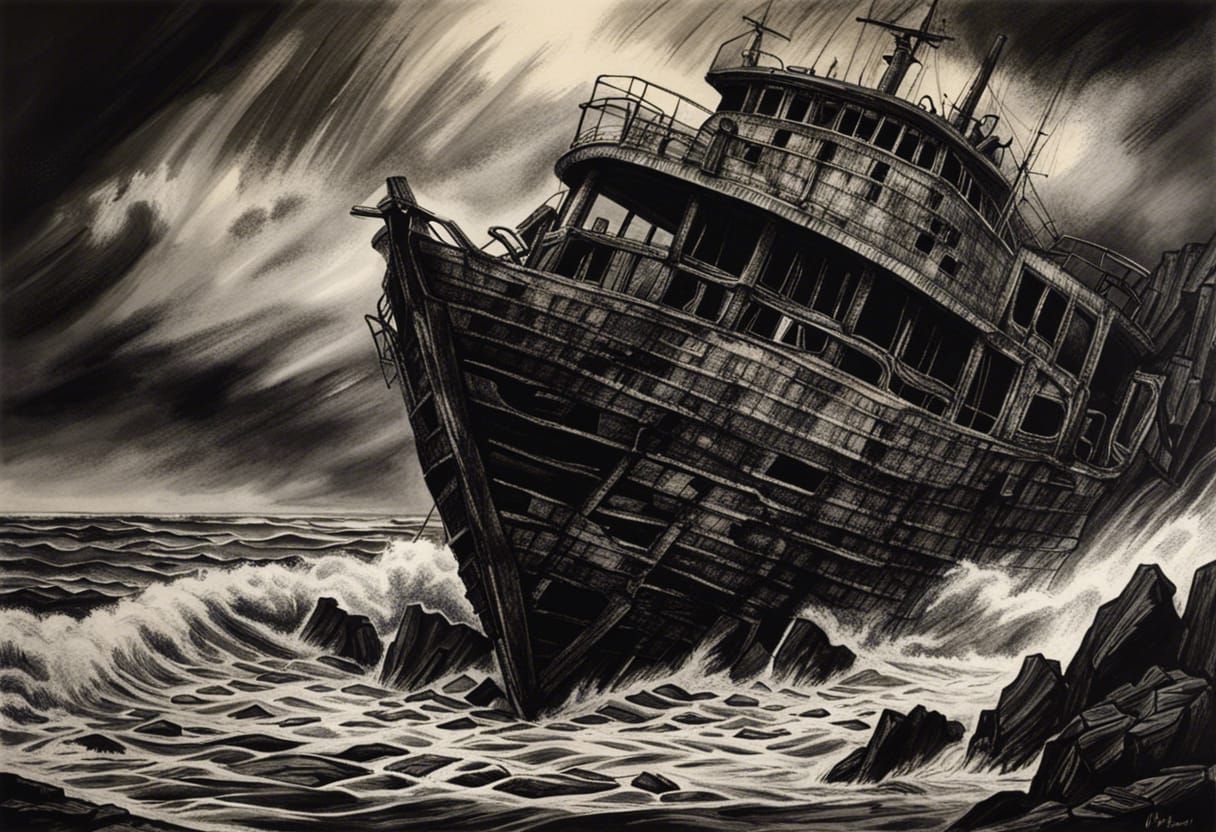This computer-generated artwork exhibits a wide vertical rectangular image set entirely in black, white, and gray tones, suggesting a stormy ambiance. The main subject is a colossal, decrepit wooden ship absent of sails, featuring an upper deck, a lower deck, and a weathered wheelhouse, indicative of its long-abandoned state. The ship leans to the right, jammed against jagged black and gray rocks that protrude from a tumultuous ocean. The background is an interpretive, stormy sky with wispy, indistinct shades of gray, white, and black. Surrounding the ship are powerful crashing waves, with a particularly massive wave surging over the stern, emphasizing the chaotic storm at sea. The scene is void of any human presence, reinforcing the derelict condition of the vessel.